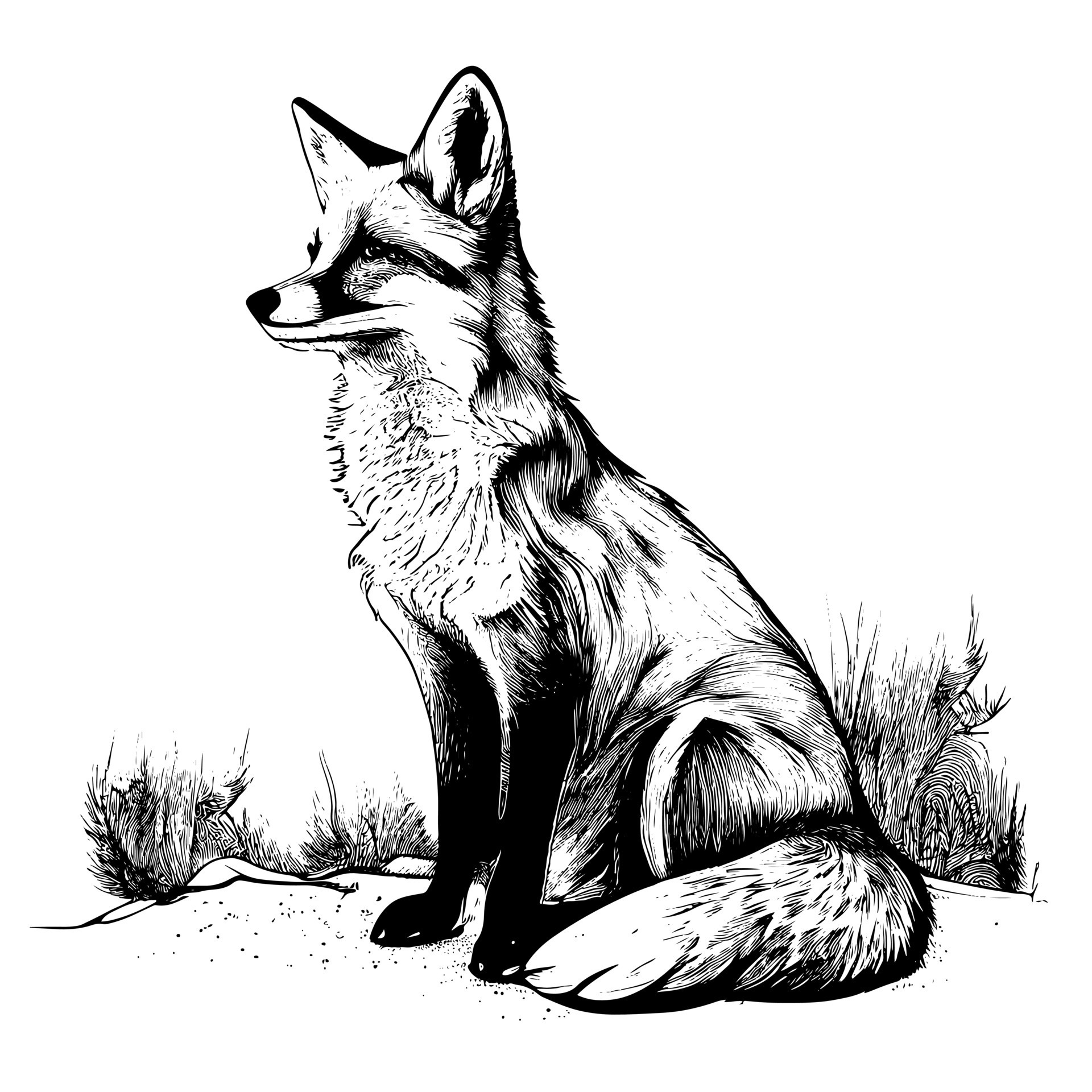This black and white drawing features a detailed depiction of a fox. The fox is positioned in profile, sitting on a ground that appears to be covered in sand or dirt, indicated by specks dispersed throughout. The fox's fur showcases intricate details, with black streaks adorning its otherwise white coat. Its jet black front legs and paws have distinct white claws. The facial features include a black nose and a black line across the top of its mouth, complementing its black-rimmed ears. The fox's tail is fluffy and prominent, curling around its body. In the background, there are scraggly plants or grasses, creating a natural setting. These plants are characterized by thin, long lines and some black swirls, adding a touch of wildness to the scene. The overall composition, rendered entirely in black and white, emphasizes the fox's striking appearance against the minimalist backdrop.